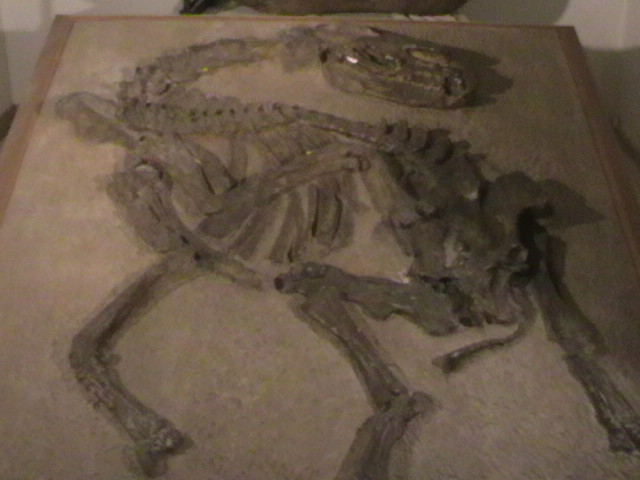The black and white photograph features a prehistoric lizard-like skeleton displayed in a museum setting. The fossilized remains are laid out on a grainy tan or cement-gray board framed in brown wood, with white walls visible in the background. The skeleton showcases a full body with a distinct head, two legs, and additional bones arranged in an S-shape. The neck bends awkwardly, positioning the head towards the spine, creating an unnatural posture. The detailed display highlights various vertebrae and limbs, capturing a comprehensive view of the ancient creature.